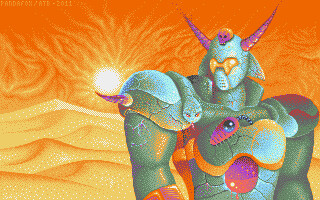A vibrant, cartoonish illustration set against a predominantly orange backdrop. The scene features a radiant sun with dynamic, multi-directional rays illuminating light orange hills below. Dominating the foreground is a towering figure adorned in an elaborate costume. The character's mask is a light blue hue with striking yellow accents around the eyes, flanked by two prominent purple horns. His massive shoulders are encased in formidable blue shoulder pads, complementing his colossal and muscular arms and chest. The intricate outfit combines shades of blue, purple, and gold, giving off a regal and powerful aura. Draped over one shoulder appears to be a blue snake, adding to the figure's imposing presence. At the center of his chest is a distinctive round purple spot, resembling an eye, further emphasizing the dramatic and mythical nature of the character.